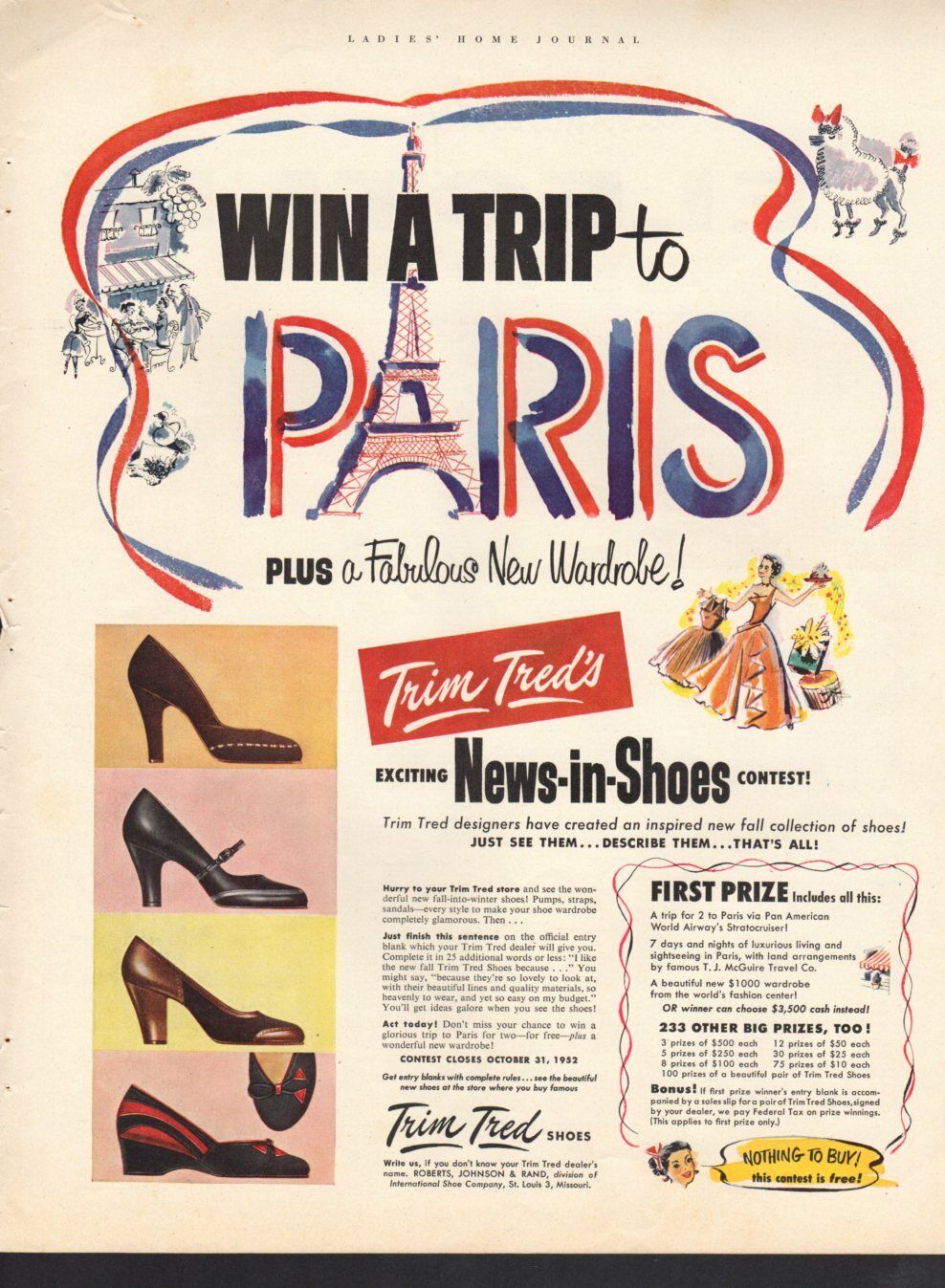This vintage advertisement, likely from a magazine like Ladies Home Journal, promotes a sweepstakes where one lucky winner can "Win a Trip to Paris" along with a fabulous new wardrobe. The title, "Ladies Home Journal," is subtly placed at the top of the poster. In this visually engaging ad, the word "Paris" creatively features the Eiffel Tower as the letter 'A', and the text is adorned in vibrant red, white, and blue colors accompanied by a ribbon banner. The contest, called the Trim Treads Exciting News in Shoes Contest, introduces an inspired new fall collection of shoes with an inviting prompt: "Just see them, describe them, that's all." The bottom half of the advertisement showcases an array of women's shoes in various colors, and details how the grand prize package includes a trip for two to Paris via Pan America's World Airways Stratocruiser. The page itself appears worn and off-white, adding to its vintage charm.